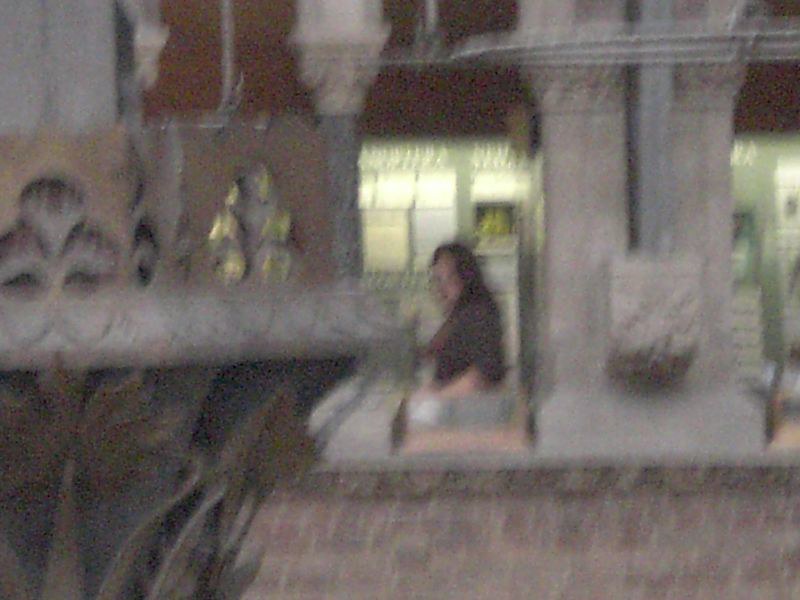This photograph, though very blurred and out of focus, captures the interior of a building that exudes a medieval aesthetic, potentially a museum or library. The architecture, which could be true stone or meticulously fabricated to mimic stone, features elaborate floral designs and a mixture of brickwork, giving an old-world feel. Positioned centrally in the image, a woman with shoulder-length brown or possibly black hair, wearing glasses and a brown, long-sleeved top with the sleeves rolled up, faces left. She appears engaged with her surroundings, potentially standing or kneeling, though her exact posture is unclear. She is amidst a collection of stone structures, including an ornate pillar on the left and a circular platform with cube-like bricks and possible lights or boxes. On the right, abstract shapes resembling shrubbery or greenery add to the setting's intricate detail. The background is decorated with columns and various shades of green, white, dark red, and black tiles, enhancing the overall mysterious and historical ambiance.